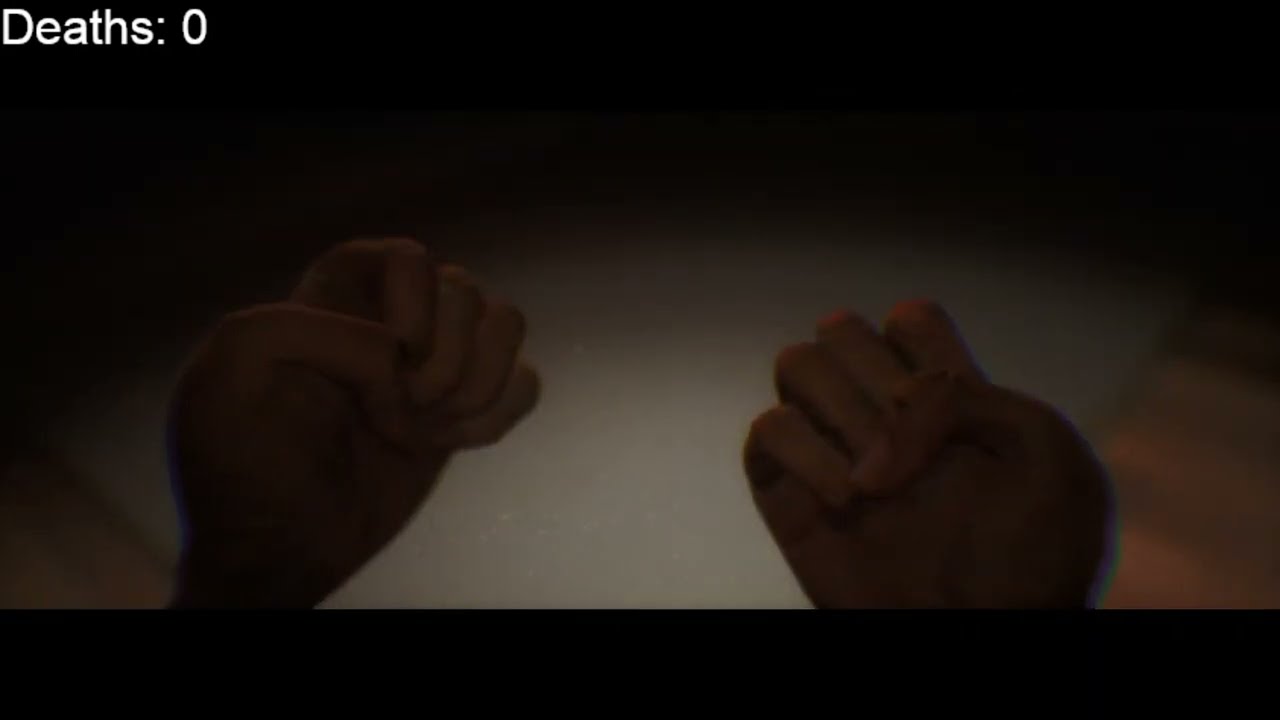This dark and blurry photograph, rectangular in shape, features a pair of hands prominently in the center. The hands are positioned as if held out with open palms, with fingers curled slightly inward and thumbs extending in front of the fingers. The quality of the photo is poor and out of focus, making detailed features indistinguishable. The background comprises a half-moon shape of white at the bottom that transitions into a dark upper portion, creating a gradient effect. There are hints of brown on the sides and some orange striped coloring. Additionally, there appears to be a faint blue aura around the hands. A thick black border stands at the top and bottom edges of the image. In the top left corner, in white print, the word "deaths" is followed by the number "0".